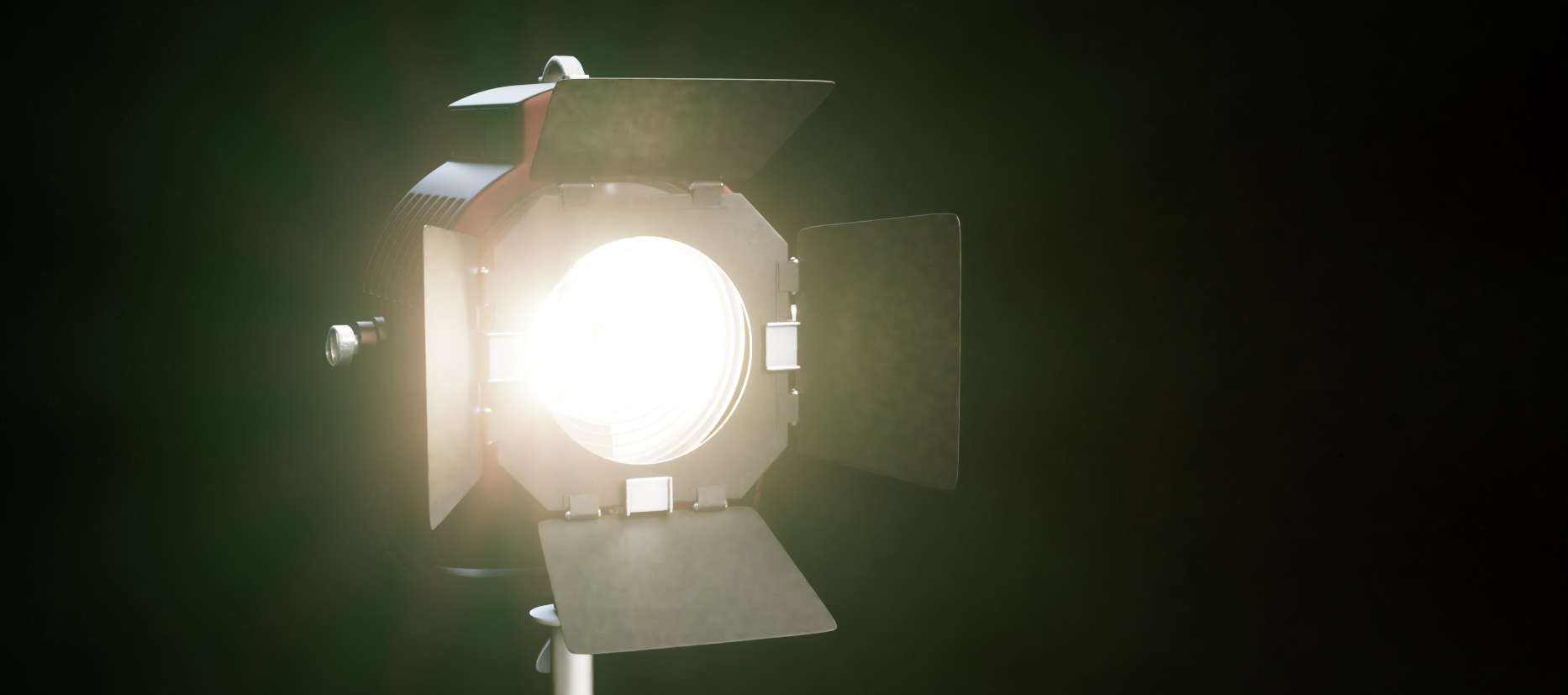The image depicts a studio light, commonly used in film production, positioned slightly to the left of center. The light features a circular, silver metal frame with an open circle at its core, where a bright yellow and white light emanates. This glowing light is surrounded by a greenish haze, set against a predominantly black background. The studio light's body is constructed from gray and black metal, with the dark metal forming the base. Four adjustable metal flaps, or panels, designed to focus the light beam, are attached around the light: one on the top, one on the bottom, and one on each side. Each flap is square-shaped and mounted on hinges, giving the appearance of a classic studio lighting setup.